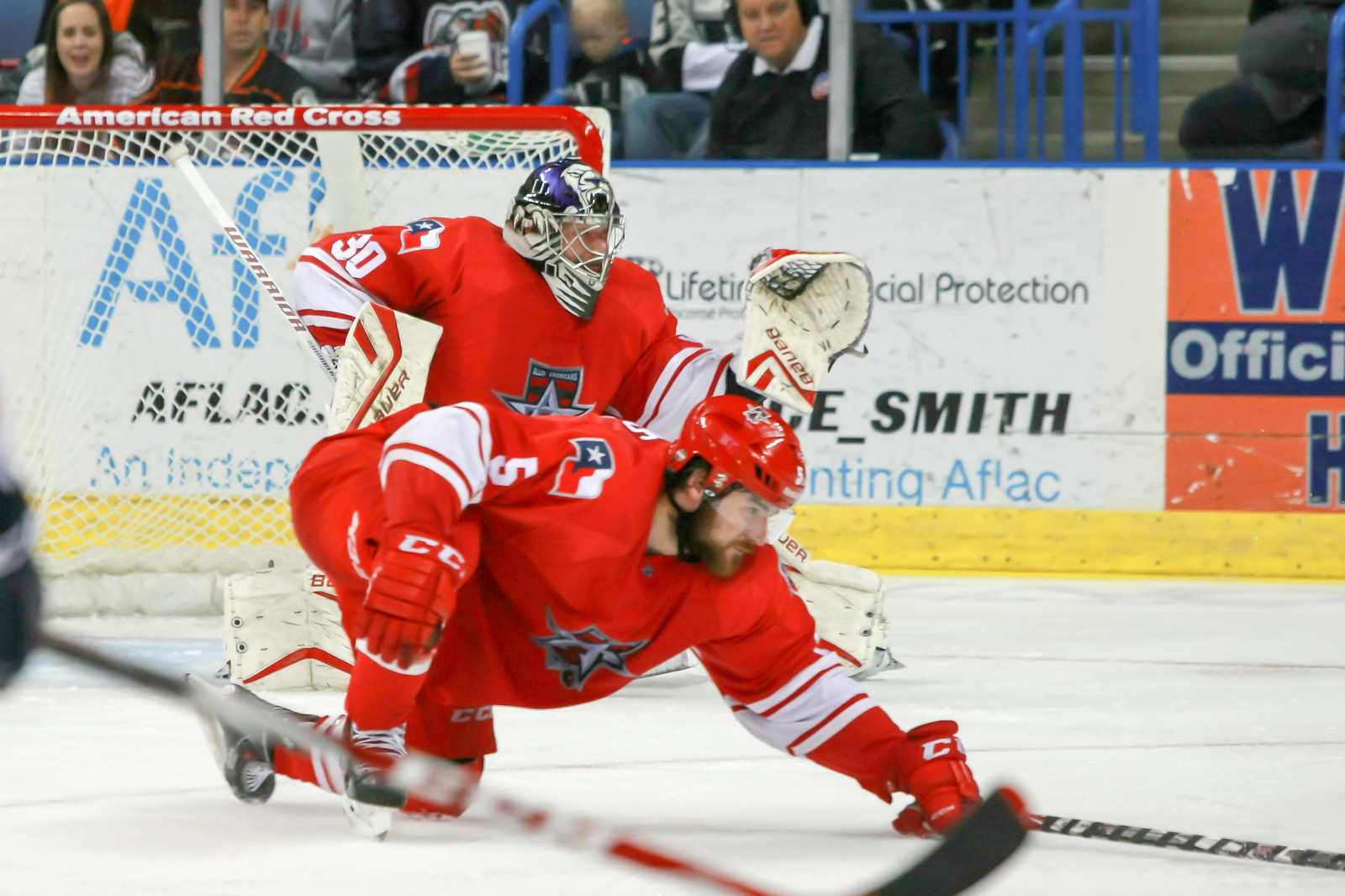The image captures a dynamic moment on an ice hockey rink where two players from the same team, donned in red uniforms and red helmets, are in the middle of an intense play. One player appears to have fallen, landing on his hands and one knee with his hockey stick on the ice, while another player, presumably the goalie outfitted with full padding and a helmet with a face mask extending down to his chin, is positioned to block in front of the goal. Scattered sticks lie on the ice, adding to the sense of action. The backdrop reveals the rink's enclosure adorned with advertisements, including those from Aflac and the American Red Cross visible on the goal itself. Beyond the rink, the stands are populated with spectators eagerly watching the game, including a small child and a fan trying to capture the moment with a camera. Though the writing on the wall is obscured by the players, the excitement in the atmosphere is palpable.